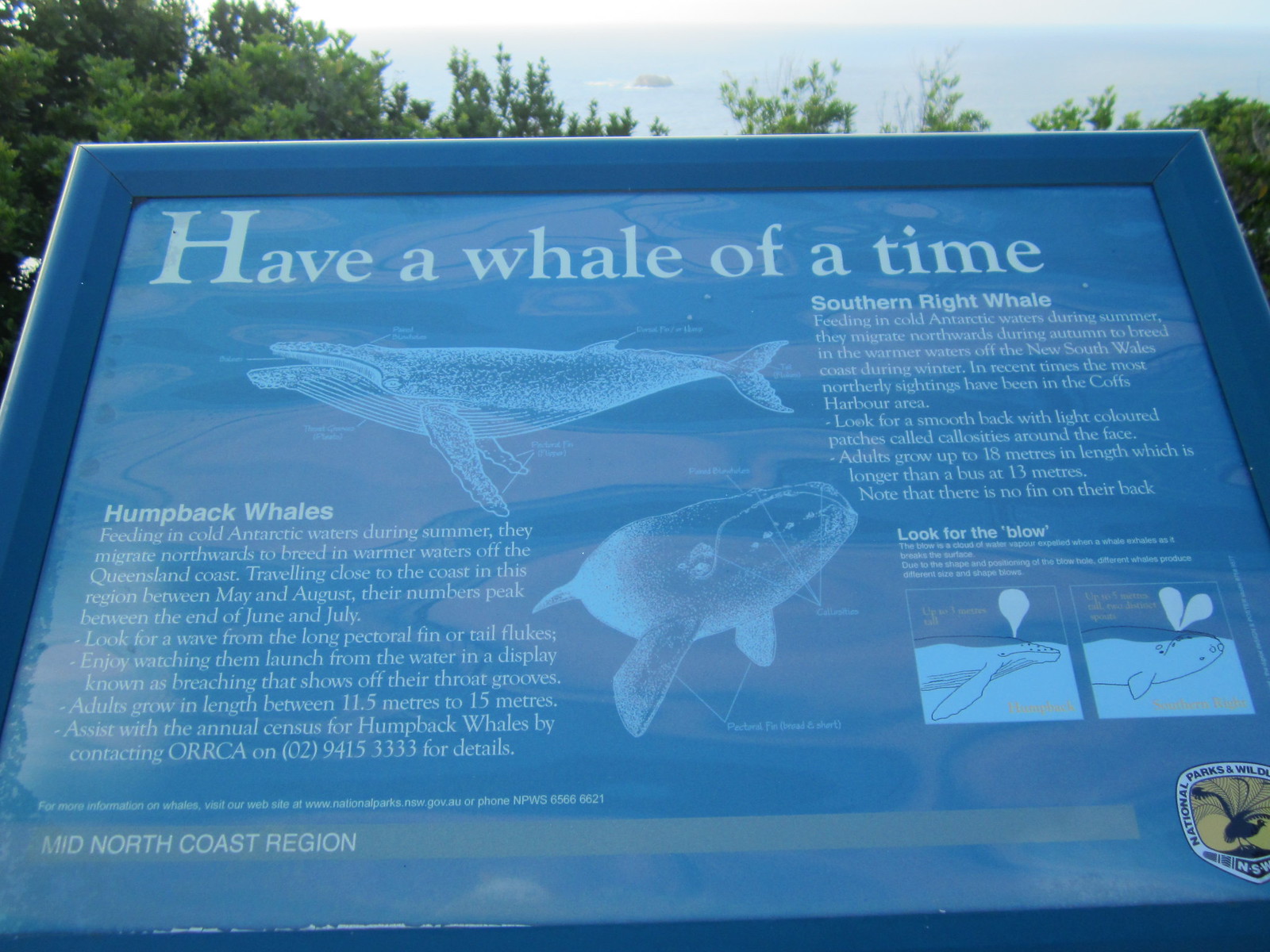The large square image features a clear, detailed photograph of an outdoor sign with a dark blue frame and background, adorned with white text and illustrations. The sign is set against a backdrop of green-topped trees and a blueish-gray, slightly blurry expanse that appears both sky and water, likely part of an aquarium setting.

Prominently displayed at the top of the sign in light-colored text is the playful caption, "Have a Whale of a Time." Below this, the sign is neatly divided into sections providing information about two types of whales. The left side is dedicated to humpback whales, featuring their name in a white heading and detailed, left-aligned text. The right side mirrors this format for the southern right whale.

Central to the sign are striking illustrations of whales. In the mid-upper section is an elongated outline of a whale, while a frontal view of another whale is positioned centrally towards the bottom. Further down, the bottom of the sign includes small square diagrams and a note to "look out for the blow," with corresponding whale blowhole illustrations, offering viewers a clear guide on identifying whale blows.

This thoughtfully designed infographic combines vibrant visuals with educational content, effectively engaging visitors at this aquatic observatory.